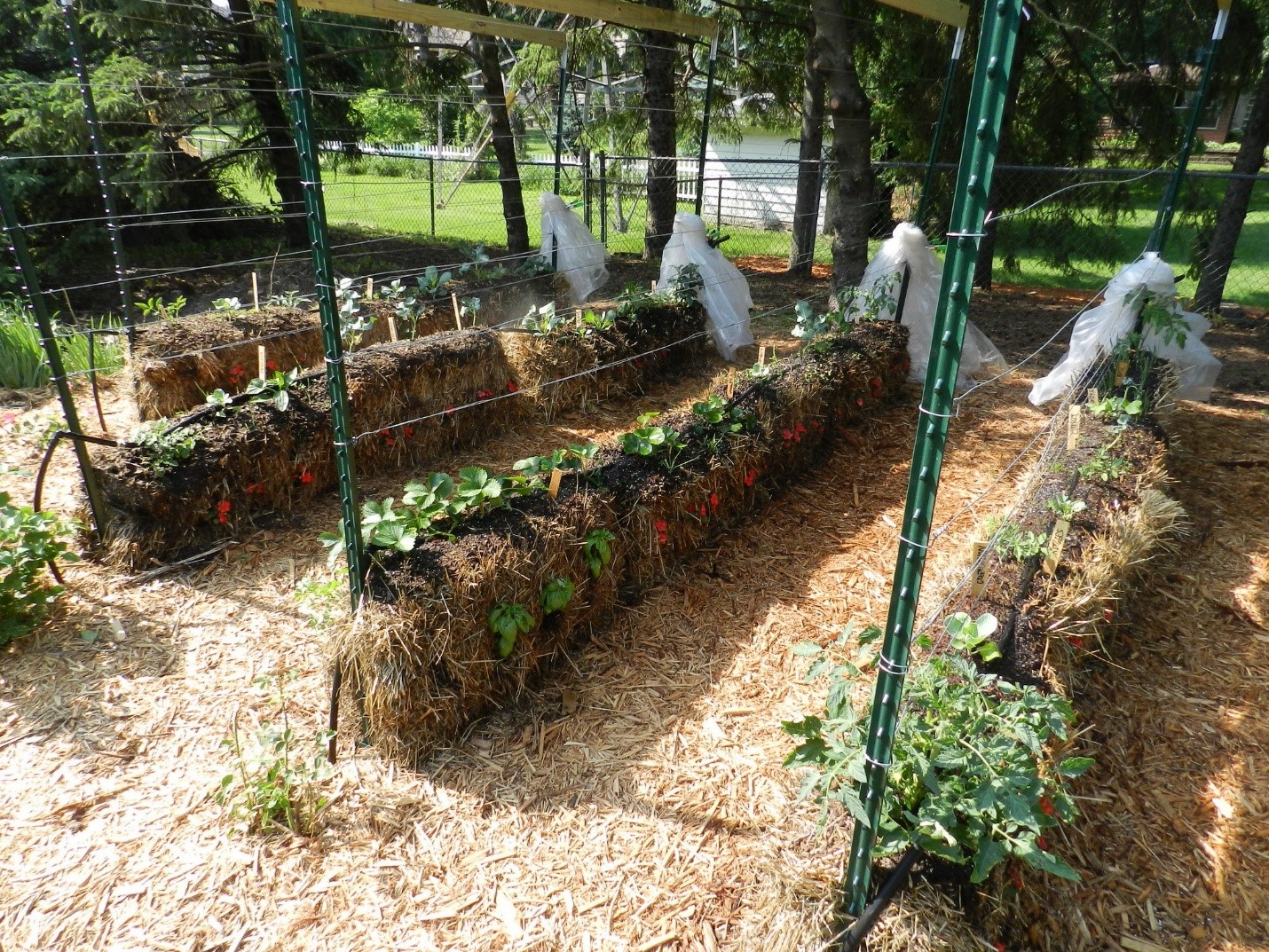This daytime photo captures a detailed view of a fenced-in backyard garden, featuring neatly organized rows of various plants. Each row is meticulously planted in hay bales or troughs, which appear to be cut lengthwise to serve as planters. The garden is subdivided with chicken wire, creating individual sections for different plants. Though it's difficult to identify the specific types of plants, there are indications that some rows might be growing berries, possibly strawberries. At the ends of the rows, there are curious white garbage bags, whose purpose remains unclear. The black chain-link fence surrounds the entire garden, while additional fencing materials are used to support trellises for climbing plants. The scene is adorned with a green lawn, trees, and a partial view of a house, all bathed in bright, sunny daylight.